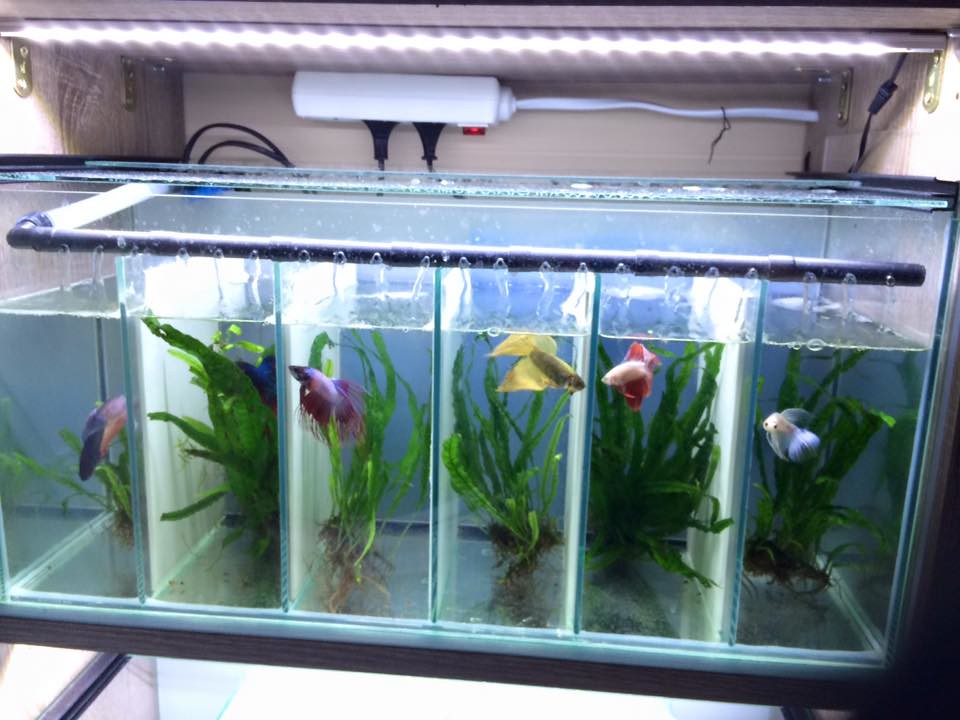The photograph depicts a large, rectangular fish tank divided vertically into six equal sections by white, opaque dividers. Each section houses a single male betta fish, each differing in color, including yellow, white, off-white with pink, purple with light pink, black with blue, and half black with light colors. Accompanying each fish is a green plant, likely seaweed or similar aquatic vegetation, contributing to a vibrant, natural-looking environment. Positioned above the tank is a fluorescent light fixture attached to a shelf, beneath which an extension cord with two items plugged in is visible. The tank, potentially used for breeding purposes, appears to rest on another piece of equipment or possibly another tank.